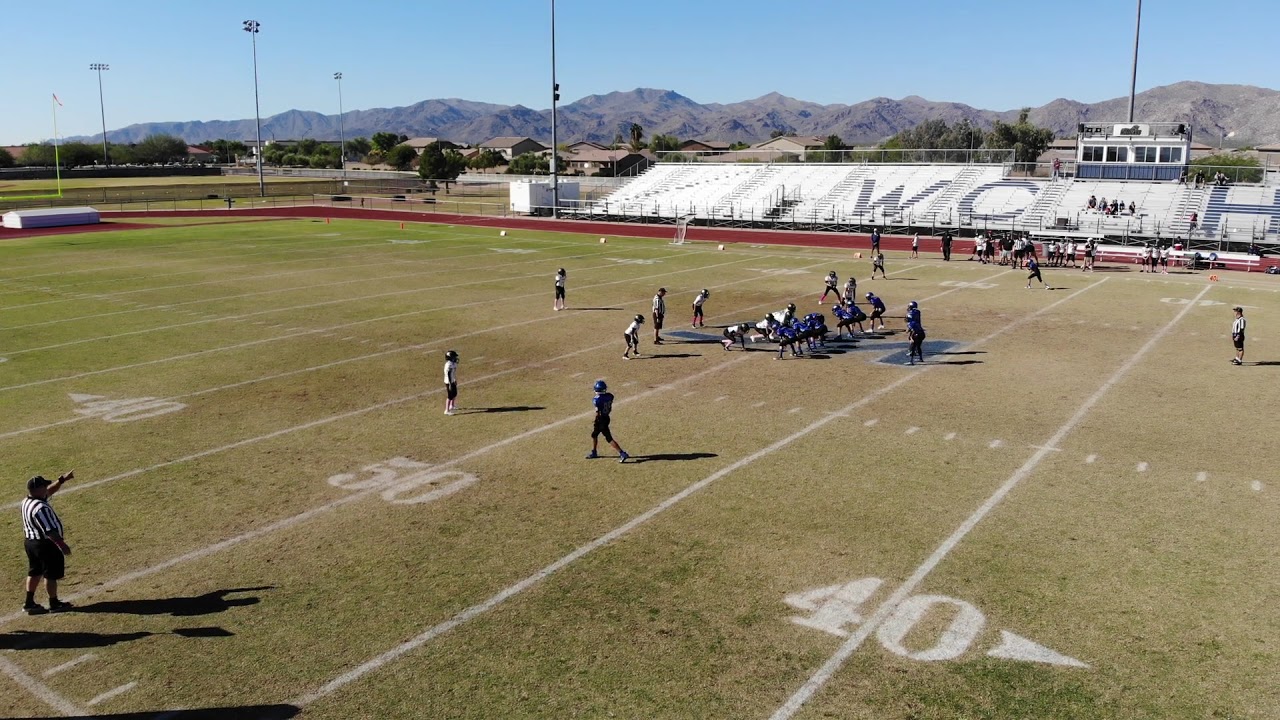This is a full-color photograph capturing a youth football game, likely in Southern California. The scene is set on a football field where the brown, patchy grass reflects the wear and tear of many games. Despite the field's condition, the yard lines are clearly marked with chalk, and the 40, 50, and 40 yard lines are visible. The game appears paused just before a play begins, with players in navy blue and white uniforms positioned near the 50-yard line. A referee, identifiable by his black shorts, black cap, and white and black striped shirt, stands in the lower left corner with his left arm extended towards the players.

The stands, painted white and nearly empty save for about five spectators, feature a prominent black "WC" logo. Additionally, a blue logo is painted on the field, partially covered by the players. In the distance, behind the field and bleachers, a neighborhood of houses is visible, along with an adjacent baseball field. Encircling the football field is a red running track. The backdrop of the scene includes mountains against a blue sky, adding to the picturesque outdoor setting.